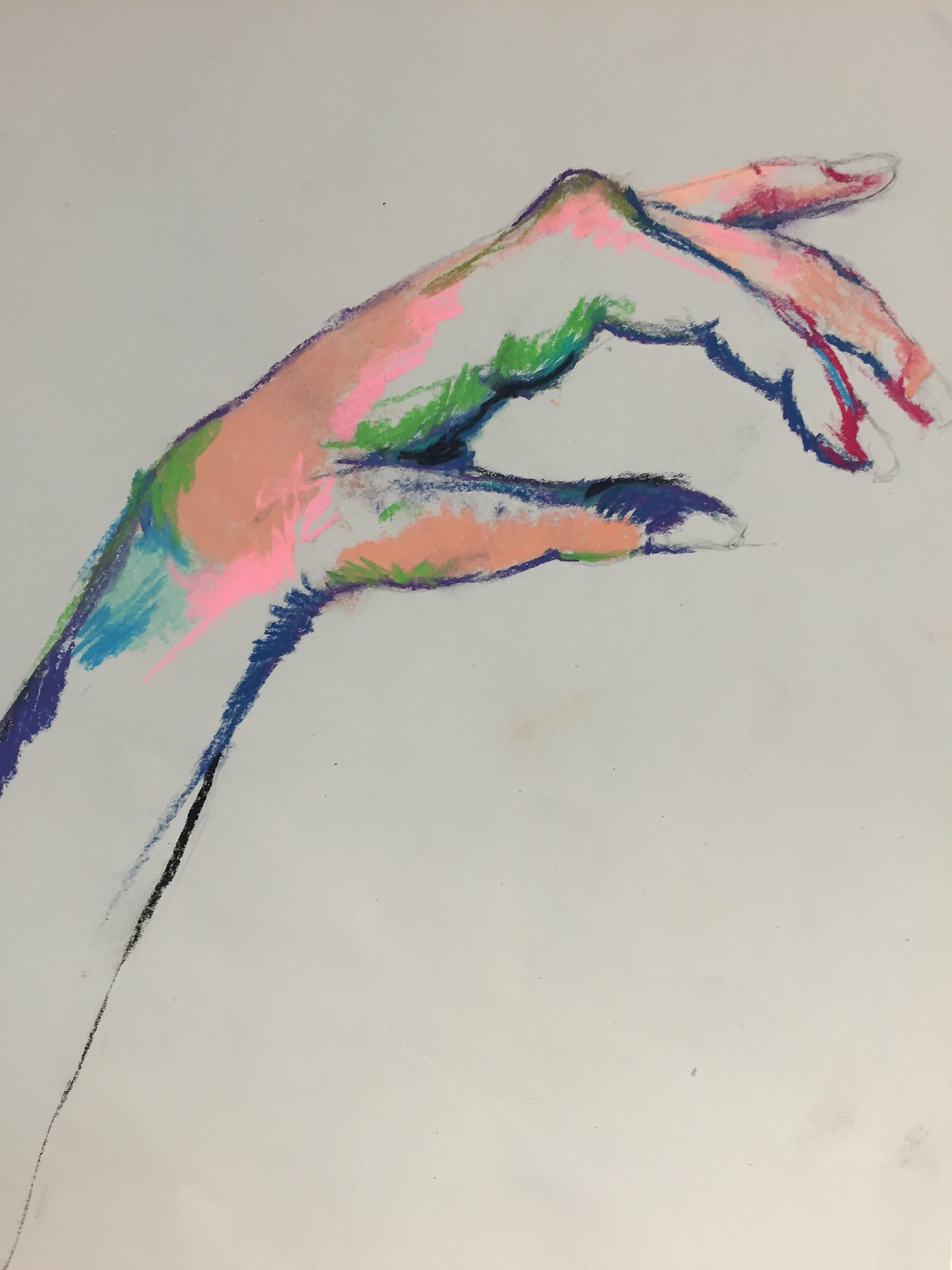This image appears to be a pastel drawing of a left hand, depicted from a side angle with the thumb in front. The hand is drawn primarily in multicolored pastels, featuring a blue outline with additional shades of pink, green, light orange, tan, aqua blue, and red. The outline has some black and dark blue shadows, adding depth to the image. The fingers are in a relaxed position, except for the pinky, which is slightly raised. The forearm extends from the bottom left of the picture, blending into the white paper or canvas that has been tinged gray due to the lighting. The fingers and thumb are vividly detailed, while the forearm remains mostly uncolored, showcasing the raw texture of the drawing surface.